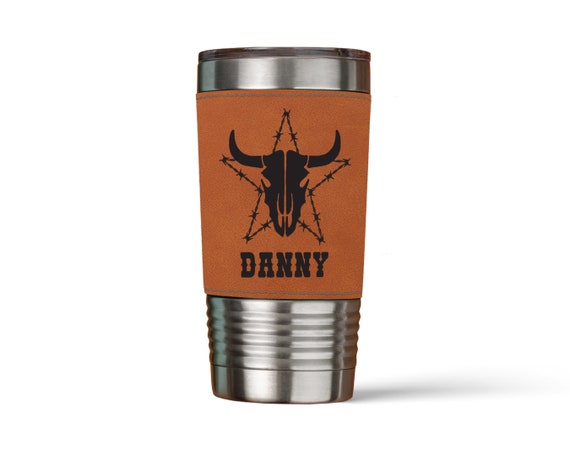This full-color promotional photograph showcases a stainless steel, insulated metal tumbler set against a stark white background. The tumbler, which casts a shadow to the right, features a two-thirds leather covering in brown. Central to the design on this covering is a stylized black steer skull, with a star made of barbed wire behind it. Beneath this striking graphic, the name "Danny" is boldly printed in black capital letters. The precise detailing suggests either a personalized or customizable product.